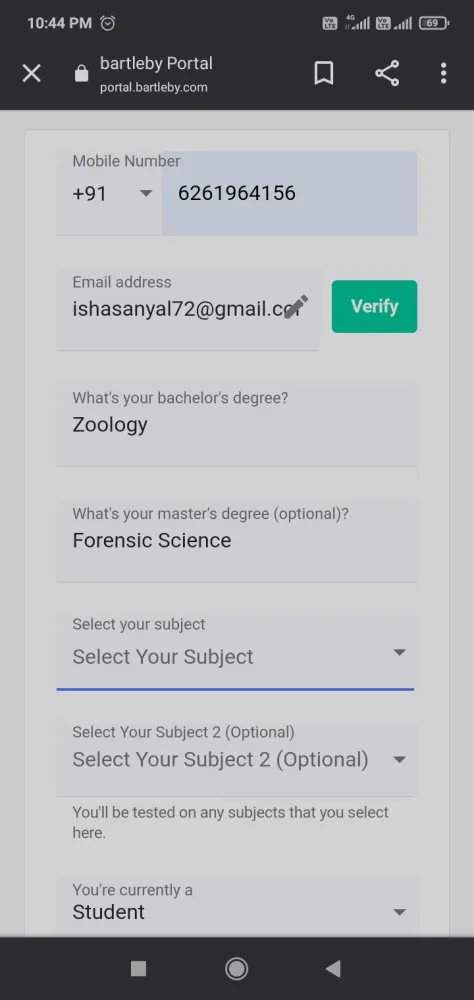The image depicts a cellphone screen at 10:44 PM, indicated by white text on a black background at the top. On the right side, there are icons showing signal strength and battery life, with the battery at 49%. Beneath the time and icons is a URL, "Bartleby Portal dot Bartleby dot com," accompanied by an "X" on the left and several additional icons on the right.

Below the URL, the background turns gray and displays a phone number preceded by a plus sign: "+91 626-1964-156", within a slightly light blue border. Further down, the gray background continues, listing an email address: "Ishanial72 at gmail dot com" with a pencil icon next to it.

A green button labeled "Verify" appears next, followed by prompts for educational qualifications: "What's your bachelor's degree?" with an answer of "Zoology," and "What's your master's degree? (optional)" with "Forensic Science" entered. The screen then asks users to "Select your subject," with a drop-down box for options, and another optional subject selection. 

At the bottom, the background is black again, framing the page.